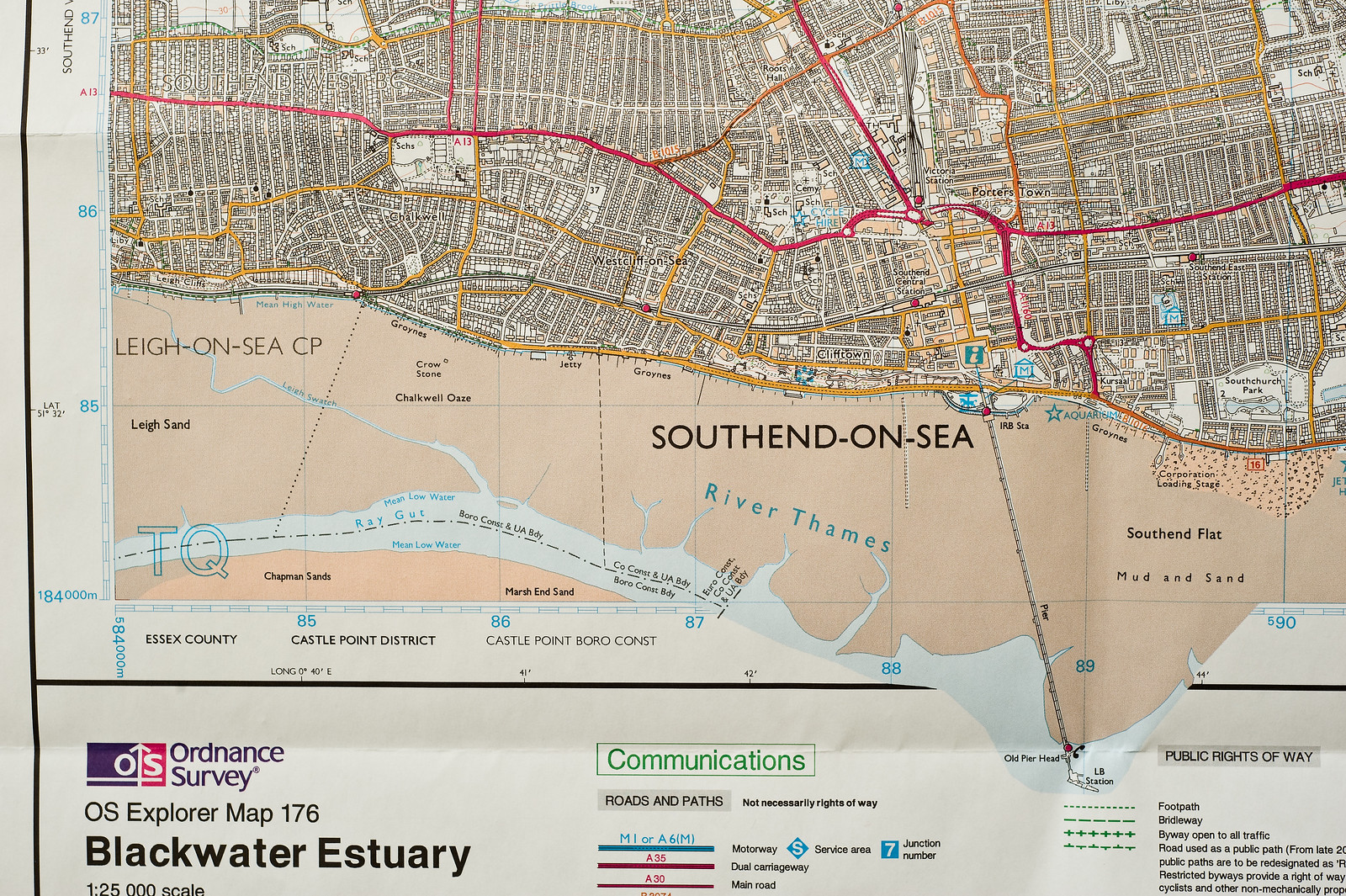This detailed photograph depicts an OS Explorer Map 176 titled "Blackwater Estuary" created by Ordnance Survey. The map, a color illustration, captures a portion of the Southend-on-Sea area near the River Thames. The intricate map shows various grids and detailed city street layouts with streets marked in red and orange intersecting lines. Additionally, orange, yellow, and black lines scattered over a city area likely denote public rights of way. The bottom left corner of the map bears the text "Blackwater Estuary" in large letters, with "OS Explorer Map 176" above it and an Ordnance Survey logo topped in red and blue. This section delineates the title and origin of the map. There is a key on the right-hand side explaining symbols used: checkered lines for footpaths, thick green checkered lines for bridgeways, green bold crossed lines for byways open to all traffic, and a unique green line resembling Arabic text denoting roads used as public paths. The background placement and creases in the top and right portions suggest that the map is hanging in a public place for easy viewing.